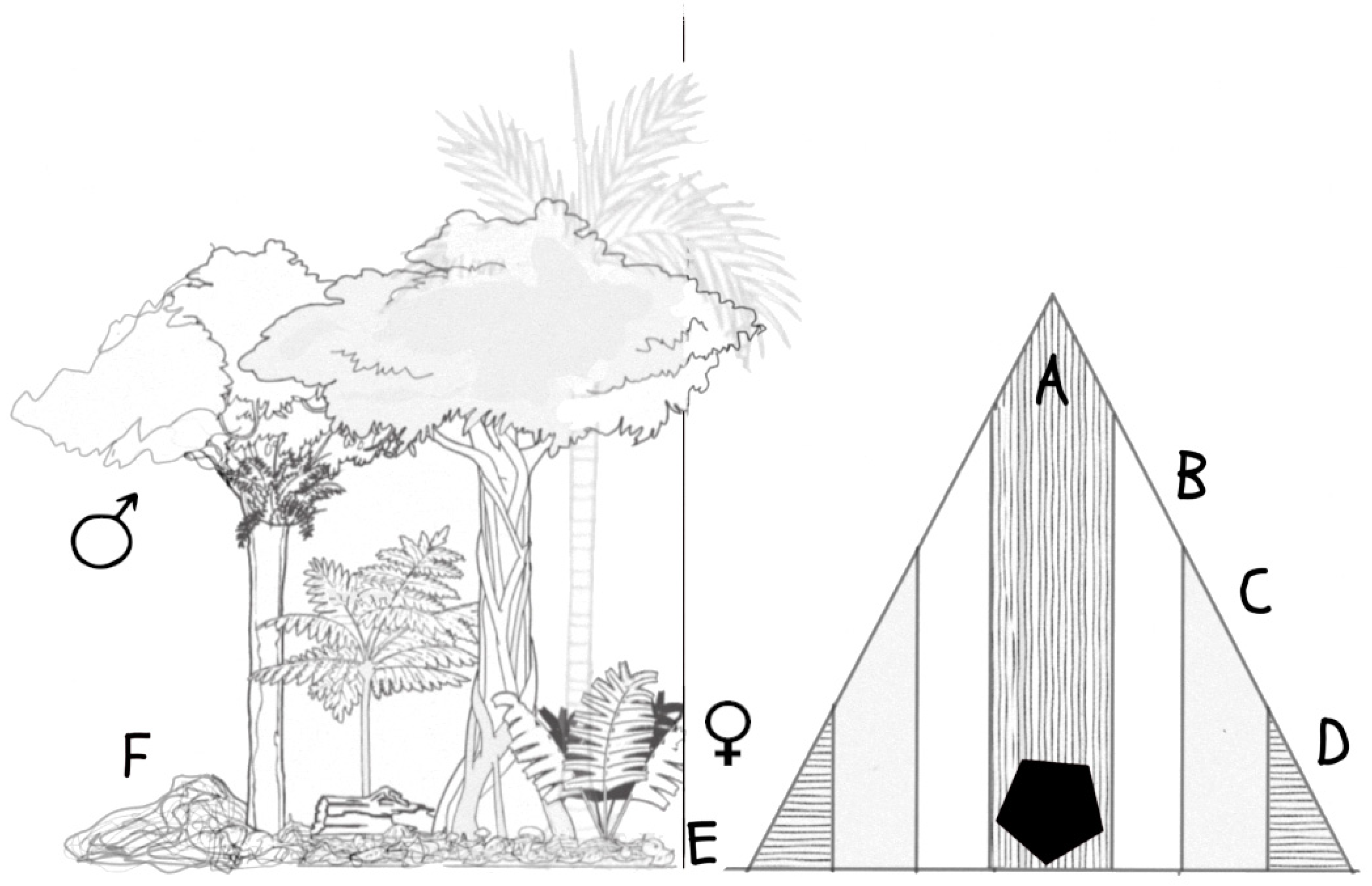The black and white diagram is divided vertically into two parts. On the left, there is a detailed sketch of a forest scene featuring various heights of foliage, including two large trees—one of which has vines—and a taller tree in the background. In between the larger trees, there are shorter trees and plants, one of which appears to be a palm tree with thin trunk lines leading up to palm leaves. Additionally, a log lies in front of one of the small trees. This side also displays the male symbol and the letter F, suggesting a connection between the foliage and a male aspect or category represented by "F."

The right side of the diagram presents a large triangle segmented into various vertical stripes and patterns. The triangle transitions from horizontal lined patterns on the outer sections, to solid sections, to vertical lines in the middle. Notably, the sections of the triangle are labeled with letters A, B, C, and D from top to bottom. Additionally, a hexagon is present along the vertical length of the diagram, suggesting a part of the categorization explained within the triangle. This side also features the letter E and the female symbol, associating these elements with a female aspect or category represented by "E."

The central column, housing the hexagon labeled A, B, C, and D, acts as a division while also connecting the two parts of the diagram, although the specific context of this relationship remains unclear.